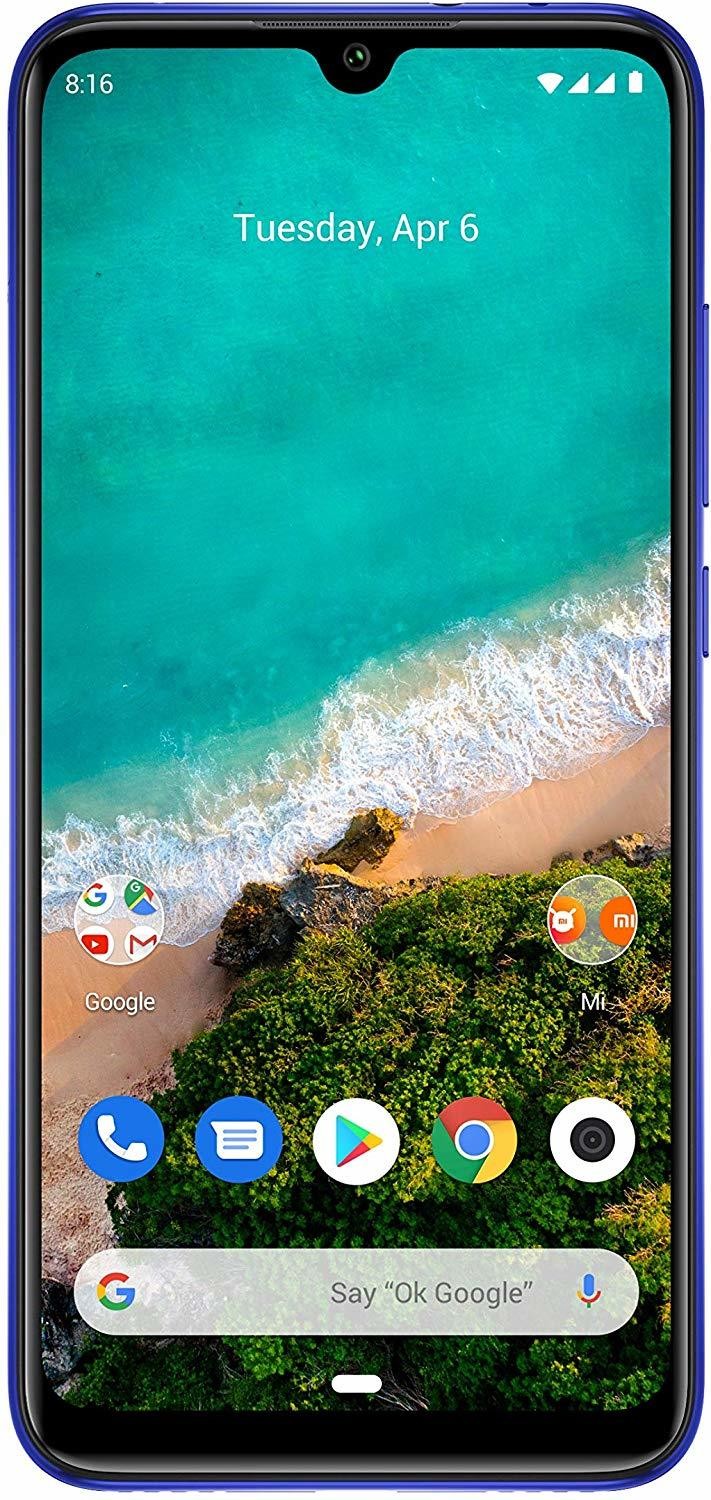The image features a smartphone prominently designed with a royal blue trim along its exterior and a black border encasing its screen. The display shows a time of 8:16 in the top center position. To the left and right of the time, various status indicators are displayed, including signal strength, battery life, cellular reception, and Wi-Fi connection.

At the top center of the phone, an integrated front-facing camera is visible. Below the time, in bold white text, the day "Tuesday" and the date "April 6th" are displayed, with "APR" notably written in all capital letters.

The smartphone's wallpaper is an aerial photograph capturing a stunning coastal scene. It shows a body of water that appears to be the ocean, meeting a sandy shore with a line of white cresting waves in between. The image also includes sections of rugged rocks interspersed with greenery that could be interpreted as grass or clusters of trees.

On the home screen, several application icons are arranged. A prominent circular icon labeled "Google" includes apps such as Google Search, Mail, and YouTube. Another circular icon with smaller orange circles and white graphics is labeled "MI" in capital letters. 

Towards the bottom of the display, additional smaller icons can be seen. Below these icons lies a Google search bar, which prompts the user to "Say, 'OK Google'" and features a microphone icon for voice searches.